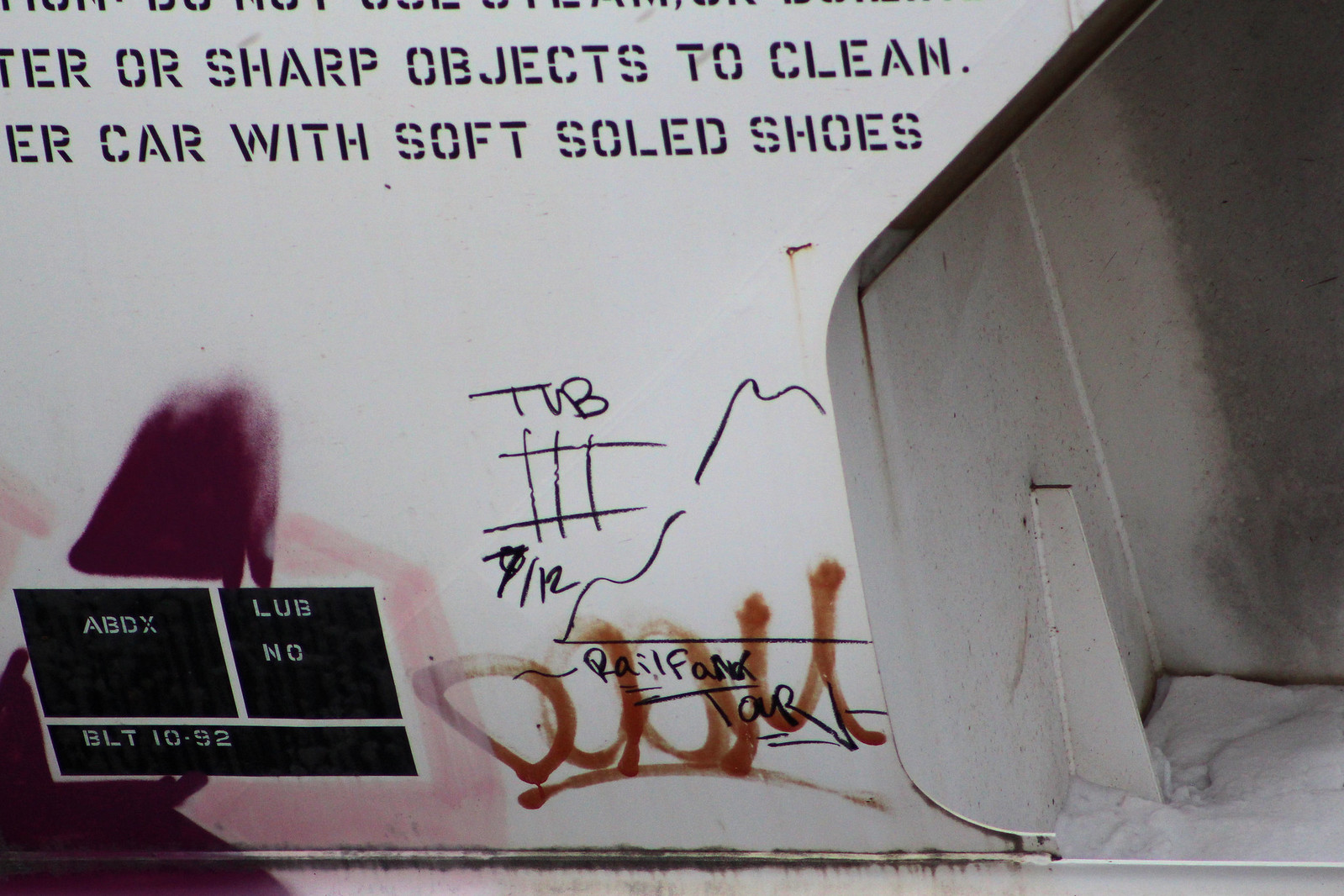The image depicts a white wall or screen with various forms of text and markings. At the top of the image, partially visible black lettering reads "or sharp objects to clean" and "car with soft-soled shoes." The background appears white with some gray streaks. Towards the bottom, there is brown, squiggly, and black graffiti that includes mostly illegible words, but "doom" is discernible in brown, underlined text. There are also marker drawings, such as "TVB," a tic-tac-toe board, and the date "7-12." On the left side, a model number "ABDXLUB number BLT 1092" appears surrounded by three separate black boxes. To the right, there's a structural beam supporting the setup. Scattered across the wall are random scribbles, including a series of black slash lines that seem to denote a count.